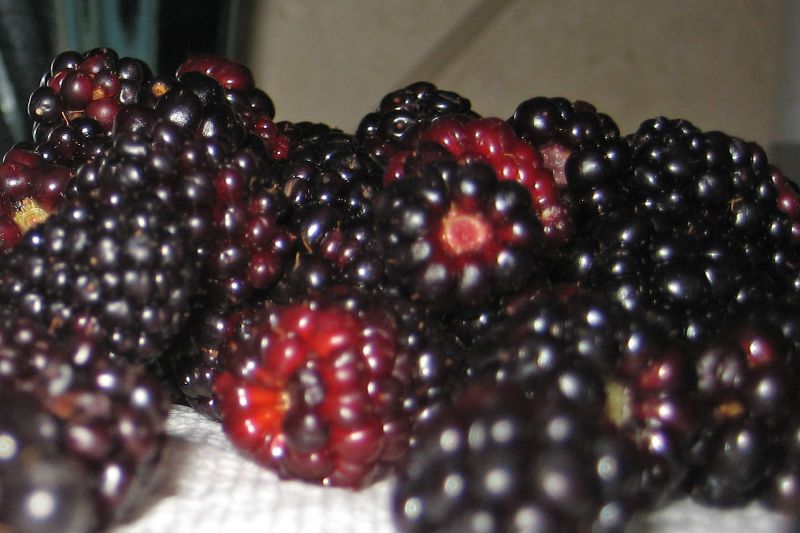This horizontal rectangular image presents a very close-up view of a clump of ripe blackberries, offering an almost abstract quality due to the varying focus across the frame. The blackberries appear significantly enlarged, with light reflecting off each of the small individual drupelets, resulting in a scattered pattern of white dots across the berries. Some blackberries reveal their central cores, adding depth to the composition. The predominantly dark purple and black berries are interspersed with a few bearing striking red hues, notably toward the left of center and in other spots throughout the cluster. This cluster of approximately twenty blackberries lies on a white, quilted surface reminiscent of a paper towel or cloth, adding texture beneath the fruit. The background includes a non-descriptive wall, with hints of a possible window or doorway in the left corner, yet it remains sufficiently out-of-focus to emphasize the artwork's main subject.